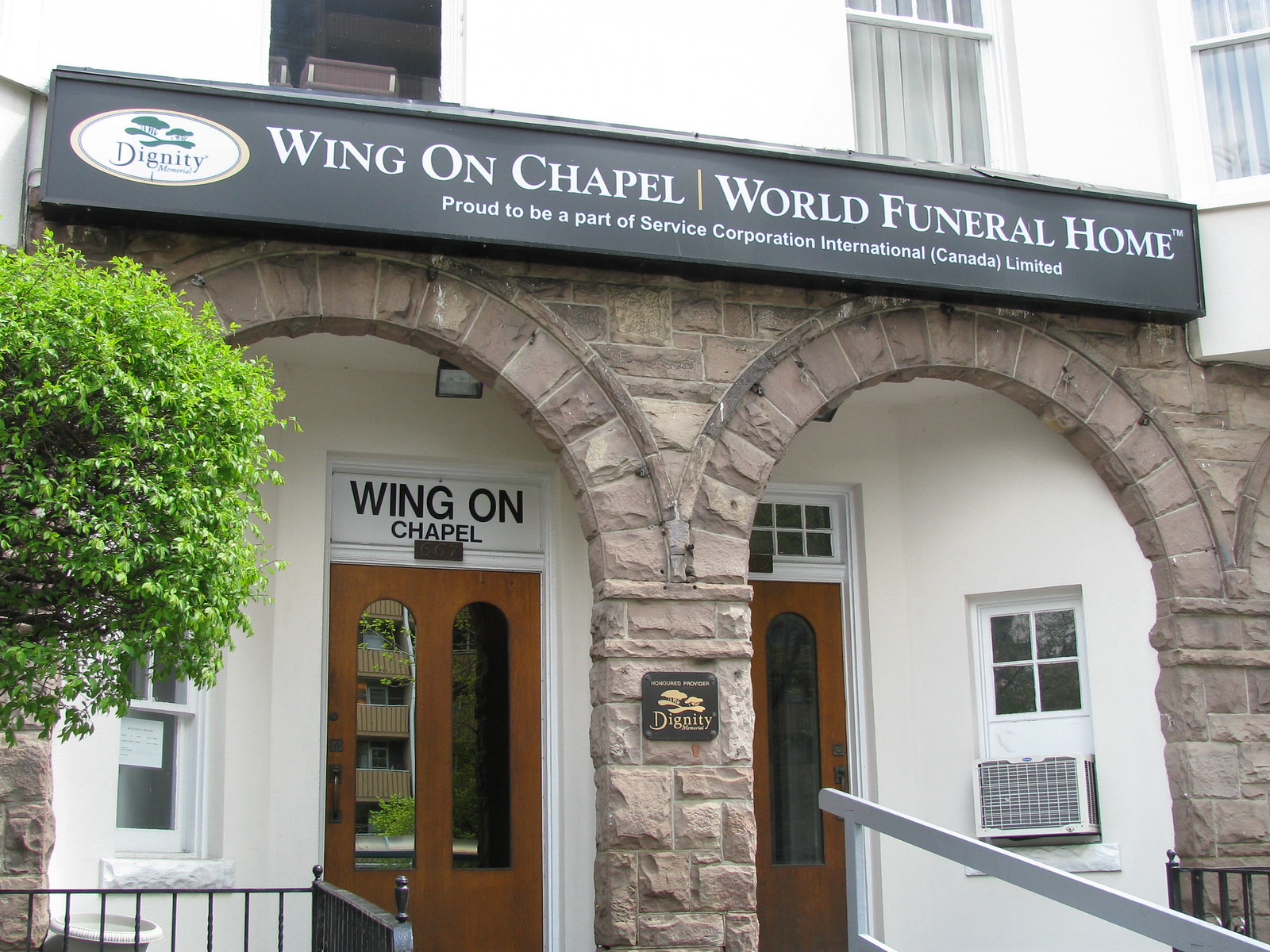The image depicts the front façade of a funeral home known as Wing On Chapel, World Funeral Home, proudly affiliated with Service Corporation International Canada Limited. The building itself is constructed with a combination of sturdy brickwork and elegant white paint that extends to the second story. Notably, the exterior features imposing arches made of gray stone that frame two prominent brown doors, each with elongated glass panels. Above the left door, the name "Wing On Chapel" is displayed, while a large black rectangular sign above the entryway proclaims the funeral home's full name and affiliation in white lettering. The structure includes several white-paned windows, one of which houses an air conditioning unit on the right side. Metal railings add a touch of practicality and style to the entrance. Additionally, a verdant green tree stands nearby, enhancing the building's dignified and serene ambiance. The image, captured in daylight, offers a clear and comprehensive view of this solemn establishment.